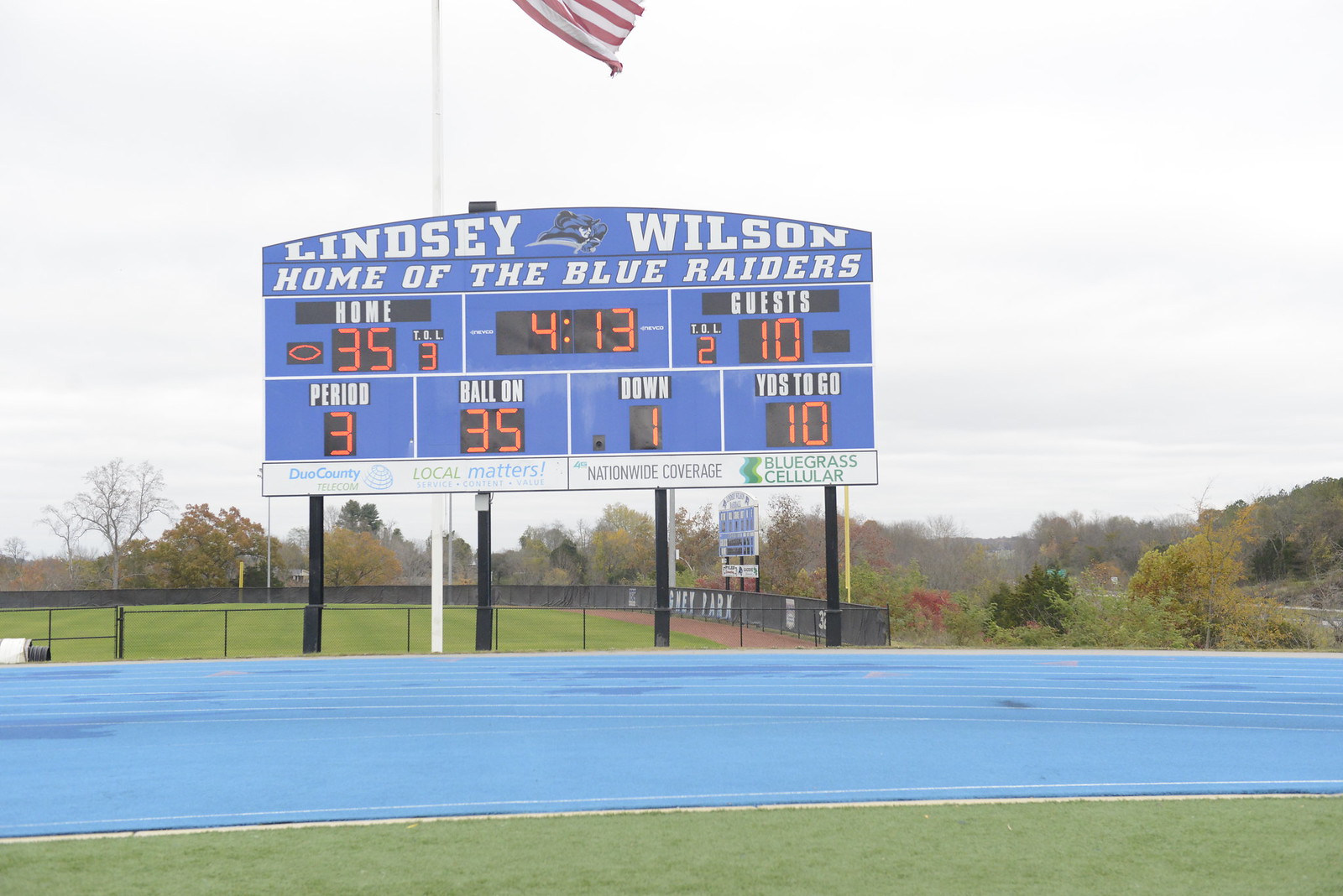This is an image of a blue football scoreboard prominently featuring white outlines to section off the information displayed. The board, titled "Lindsay Wilson Home of the Blue Raiders," stands against a cloudy backdrop with a white flagpole visible near it. The scoreboard is adorned with the school mascot at the center and the details of the game are as follows: the home team leads with a score of 35, having 3 timeouts left (TOL 3), while the guests have a score of 10 and 2 timeouts remaining (TOL 2). The game is in the third period with 4 minutes and 13 seconds left on the clock. The board also indicates that the ball is on the 35-yard line, it is the first down, and there are 10 yards to go. Below the game information, there is a section that displays sponsor names such as Bluegrass Cellular, Nationwide Coverage, and possibly a local mattress company. In the background, beyond the scoreboard, there is a glimpse of a baseball field enclosed by a black fence and topped with a blue track, adjacent to some trees. The photo appears to be taken from the 50-yard line of the football field.